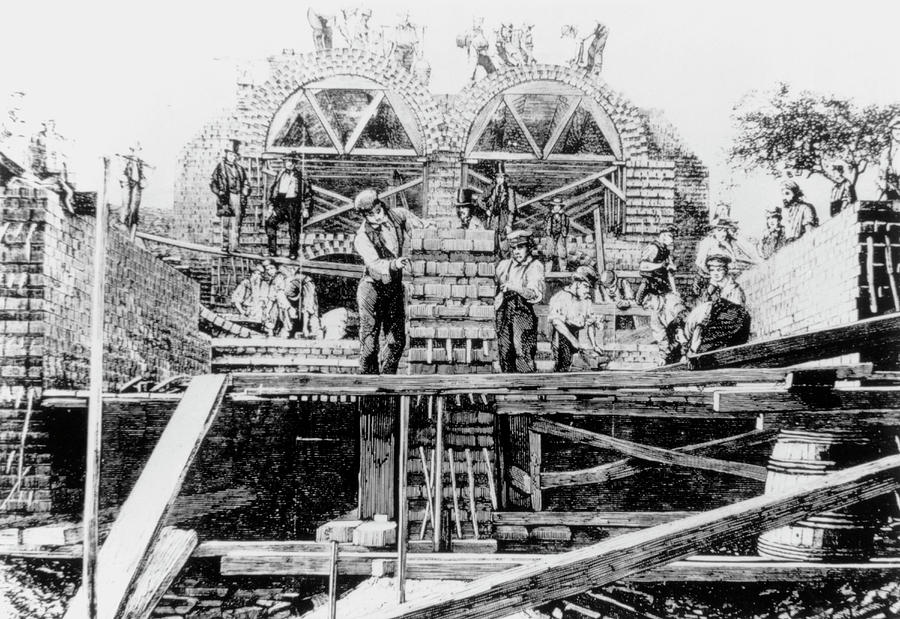This detailed black and white drawing depicts a bustling construction site from a bygone era, possibly the construction of a large building or house. The scene is filled with over twenty workers actively engaged in various tasks. Many of these workers are situated on wooden planks and scaffolding, arranging bricks to build the structure's walls. The left and right walls appear to be largely completed, showcasing intricate circular designs and arched windows at the top. In the foreground, several workers are seen adjusting bricks and moving materials, while others stand on different levels of scaffolding in the background. Notably, two men in top hats and jackets can be observed on the left side, adding a touch of period-specific detail to the scene. Scattered around are numerous stacks of bricks and wooden logs, along with a barrel, contributing to the authentic construction ambiance. A lone tree behind the right wall adds a natural element to the otherwise busy scene, with a grey sky overhead. This highly detailed illustration captures the essence of a historical construction site with remarkable accuracy.